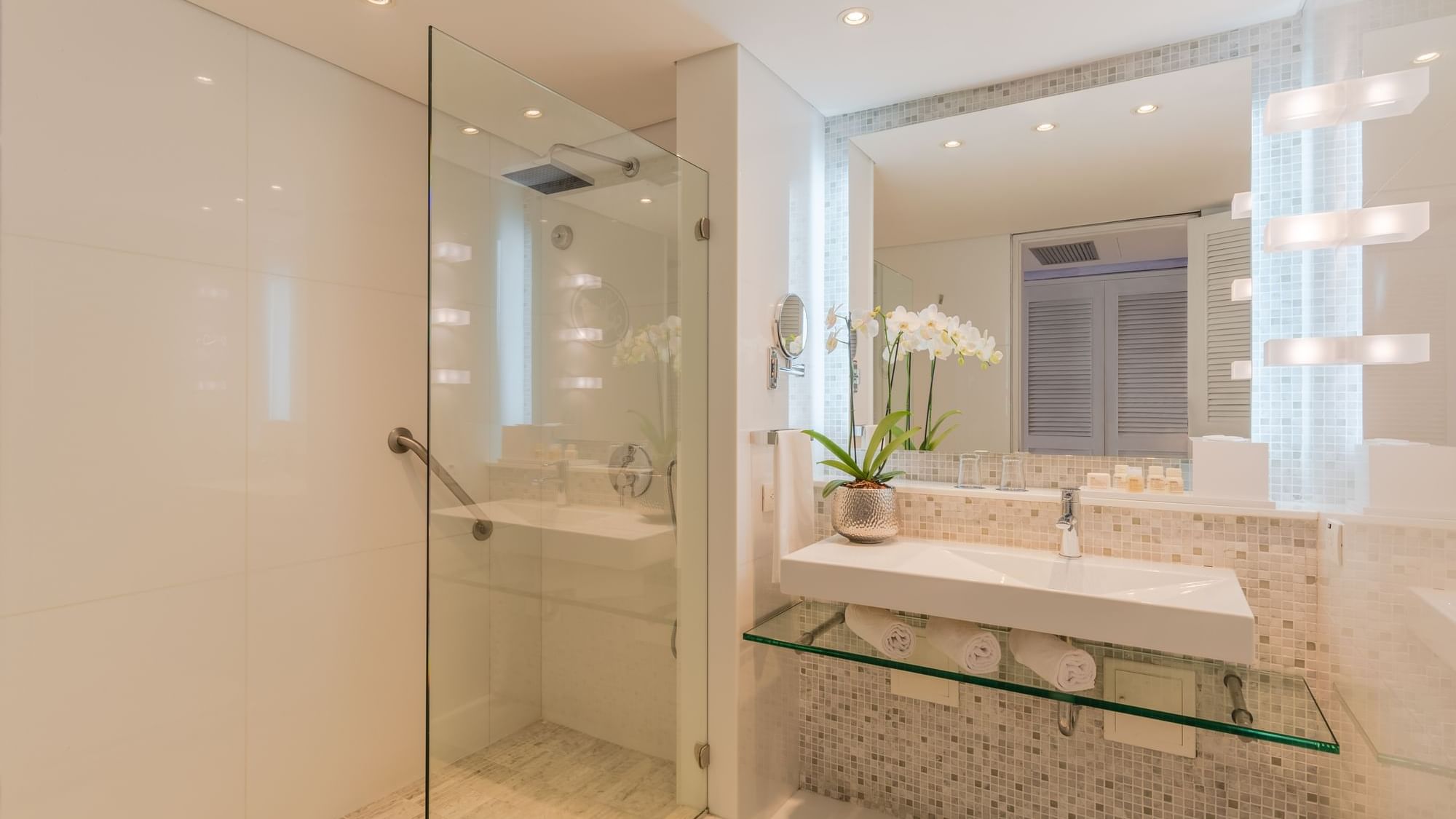This image depicts a meticulously designed corner of a modern hotel bathroom. Dominated by clean lines and a minimalist aesthetic, the bathroom features predominantly white decor interspersed with clear glass elements. On the left side, there is an open walk-in shower with a sleek clear glass partition and silver knobs for controlling the water, accentuated by a ceiling-mounted rain showerhead. Adjacent to the shower is a broad horizontal rectangular mirror flanked by lights on either side.

Below the mirror, a white vanity with brown and white tile accents supports a flat rectangular sink. The sink area is pristine, with no items cluttering its surface. Beneath the sink, a wide, clear glass shelf holds neatly rolled white towels, enhancing the bathroom’s clean and organized look. A small green potted plant adds a touch of natural color to the space. The overall arrangement and the reflective surfaces, including glimpses of a closet door in the mirror's reflection, suggest an upscale, serene, and spacious bathroom likely found in a hotel setting.